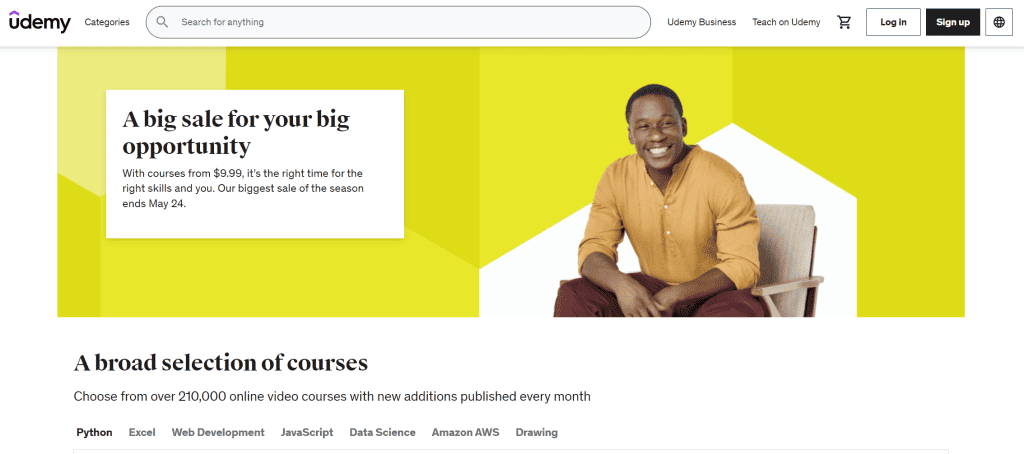The image is a detailed screenshot from the Udemy website, showcasing its interface and a promotional banner. In the upper left corner, the Udemy logo is displayed in lowercase black text with a distinctive purple arrow pointing upwards over the "u". Adjacent to the logo, there is a prominent search bar spanning almost half the width of the screen, allowing users to search for courses.

To the right of the search bar, there are several options: "Udemy Business," "Teach on Udemy," a shopping cart icon, a login button, and a sign-up button.

Below these elements, the centerpiece of the image is a vibrant promotional banner against a yellow background. In this banner, a young black man in his 20s or 30s is seated and smiling at the camera. He is dressed in a mustard-colored button-up shirt with brown pants, with his sleeves rolled up to his elbows, giving a casual yet professional appearance.

Accompanying the image is a bold text box with a promotional message: "Big sale for your big opportunity. With courses from $9.99, it's the right time for the right skills in U. Our biggest sale of the season ends May 24th."

At the bottom of the banner, additional text highlights Udemy's vast selection of courses: "Choose from over 210,000 online video courses with new additions published every month."